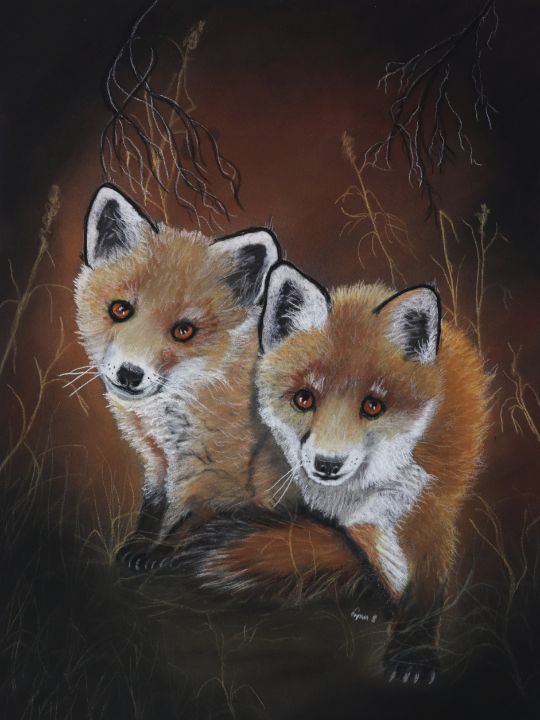This painting captures two young red foxes, their curious expressions directed straight at the viewer. The fox in the foreground, a lighter shade of red with a white-tipped tail, seems almost scared, while the fox behind has a more neutral demeanor. Both foxes share striking features: reddish-orange fur, white snouts and chests, brown eyes with white ear tips, and brown noses. Their paws, tipped with black claws, are slightly visible. They appear to stand amid a field, though the background blends into darker tones with scattered imagery of roots, dead grass, and branches, creating an ambiguous, twilight setting. The subtle artist's watermark lies unreadable within the composition, adding a layer of mystery to the artwork.